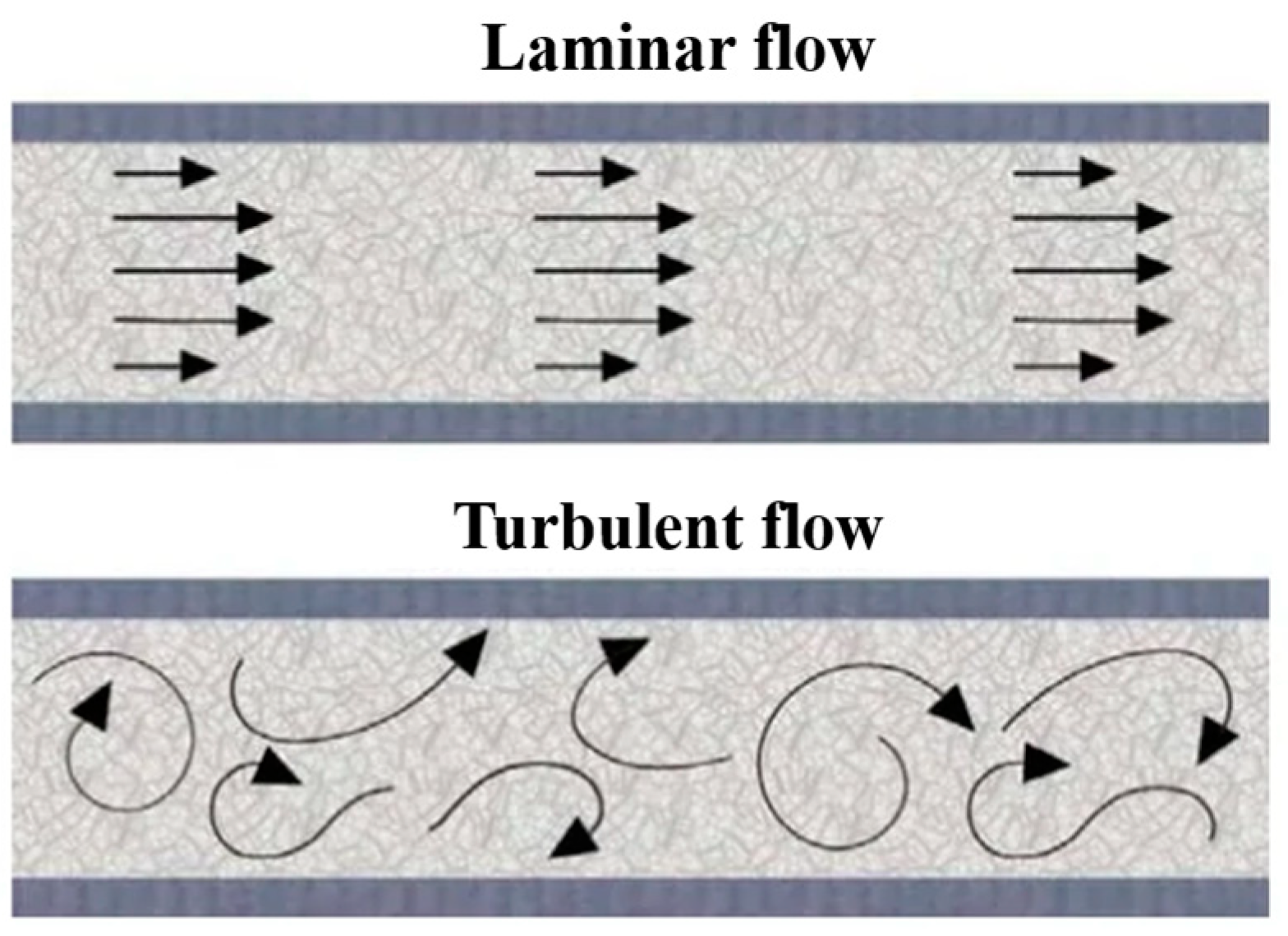The image is a detailed scientific diagram illustrating two types of fluid flow. The top section is labeled "Laminar Flow" in black text and features a rectangular diagram with gray strips at the top and bottom. Within this rectangle, there are three rows of five black arrows pointing straight to the right, symbolizing uniform flow. The background within the rectangle is a muted gray, representing the fluid medium.

Below this, the bottom section is labeled "Turbulent Flow" in black text and contains a similar rectangular diagram with gray strips. However, in this section, the seven black arrows are depicted in chaotic, swirling patterns, symbolizing disordered and unpredictable flow. The background around both sections is white, creating a clear contrast with the black arrows and text. The diagram includes subtle colors like light green, a tinge of pink, and white lines, adding a nuanced representation of the fluid dynamics involved.